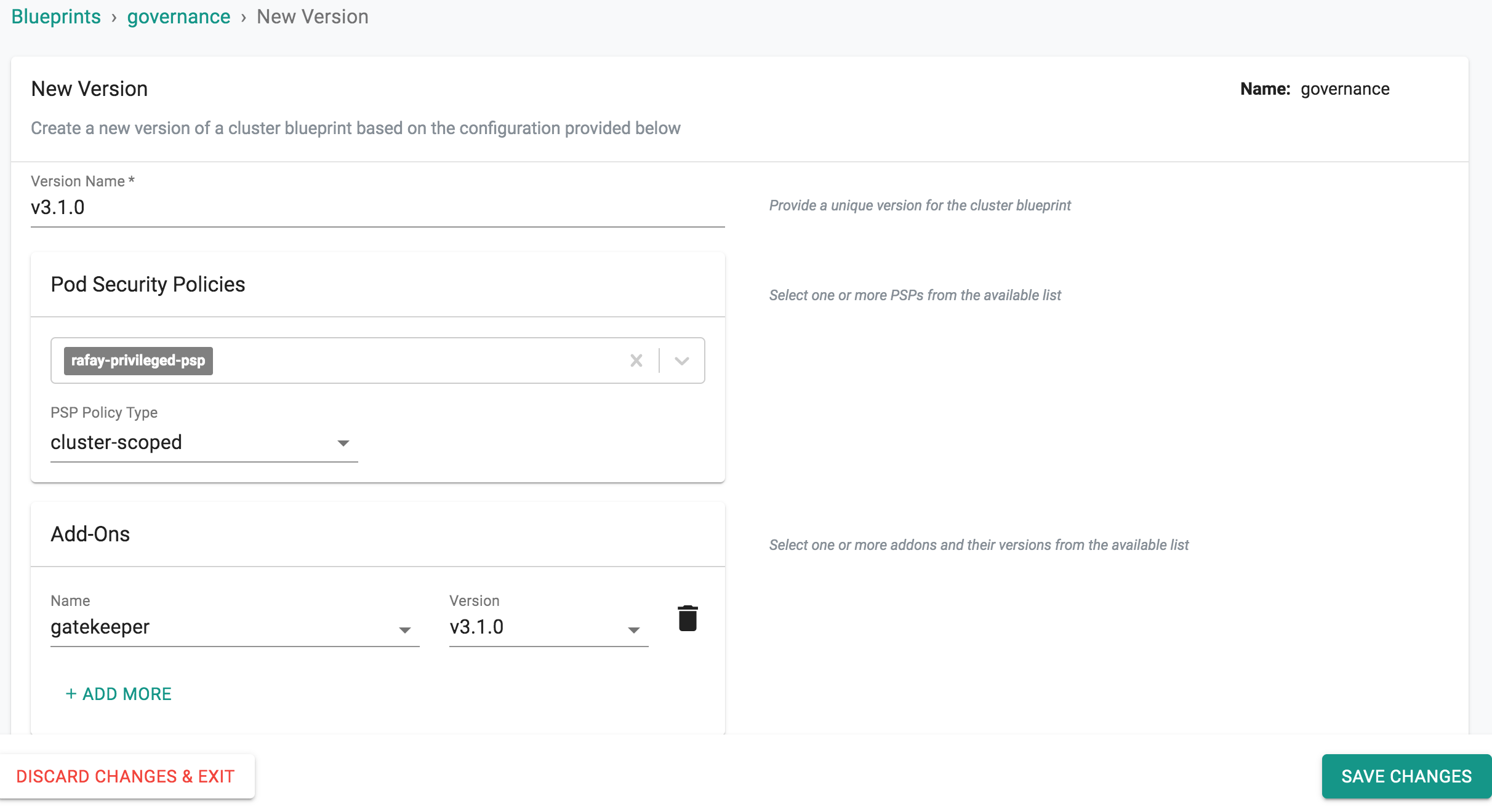A well-organized user interface for updating cluster blueprints is displayed. The upper-left section features blueprints with an arrow pointing to the right labeled "Governance," followed by another arrow pointing to "New Version." Below this, options are provided for either creating a new version of the cluster blueprint based on the existing configuration or opting not to create a new version at all.

On the right side, a detailed form starts with a section labeled "Name" and "Governance." Beneath this, fields for inputting the version name (e.g., "v3.1.0") and selecting pod security policies (PSPs) are available. The current PSP, labeled "rafay-privileged.psp," is in a dropdown bar with a removable option marked by an 'x'. There is also another dropdown for the "PSP Policy Type," set to "Cluster Scoped."

Additional configuration options include a section for "Add-ons" where users can select an add-on name (e.g., "Gatekeeper") from a dropdown menu, along with specifying its version, also "v3.1.0," from another dropdown. Beside these selections, there is a trash can icon for removing add-ons, alongside a green "+ Add More" button to incorporate additional add-ons.

At the bottom of the interface, a red button labeled "Discard Changes and Exit" allows users to abort changes. Instructions on the right side guide users to provide a unique version name for the cluster blueprint, select one or more PSPs from the listed options, and choose the required add-ons and their respective versions.